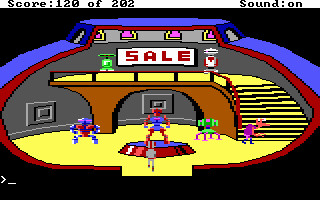A detailed caption for the image might read:

"In this digital game scene, the player has a current score of 120 out of 202, with the sound feature turned on, as indicated at the top of the screen. The game's setting is against a stark black background, highlighting a blue spaceship that appears partially cut open, revealing intricate interior details. Pink lights illuminate the top contours of this vessel. Dominating the foreground is a grand, slightly spiraling staircase that exudes a foreboding presence. This staircase curves upward to an elevated landing area, prominently marked with a large 'SALE' sign. At this landing, two robots are positioned: one with a green chassis and another in red and white hues. Near the bottom of the scene, two digital figures are present; one is positioned inside a circle, while the other stands off to the side. Adding to the scene's ambiance is a lone green chair placed near the bottom left corner."